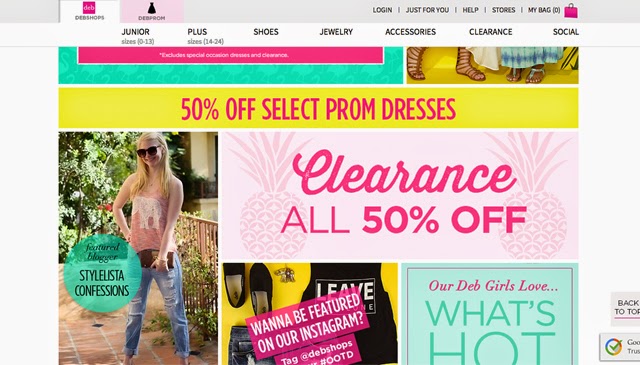The homepage of DEB Shops, a comprehensive website dedicated to women's fashion, features an array of categories including juniors, plus sizes, shoes, jewelry, accessories, clearance items, and social content. Above these categories, users can find options for login, personalized recommendations under "Just For You," help resources, and store information. Also prominently displayed is the shopping cart, symbolized by a pink emoji bag icon.

The website offers two distinct shopping platforms: DEB Shops and another variation called Deb From, with the current view set to DEB Shops. The DEB Shops logo, a small pink icon with "DEB" written in white, is located at the top.

Below the logo is an image of a smiling girl dressed in jeans and a white tank top featuring a white elephant print. The setting appears to be outdoors, with a sidewalk and railing in the background. Adjacent to her image is a green circular badge labeled "Featured Blog, Stylist Confessions."

Further up, a pink banner with a yellow outline announces a "50% Off All Selected Prom Dresses" promotion. To the right of the girl, in a script-like font, the word "CLEARANCE" is displayed in pink, with "ALL 50% Off" in bold capital letters directly below it. The page is accented by several pink pineapple watermarks.

Below these elements, a tilted box inquires if users want to be featured on Instagram, surrounded by images of shoes and what appears to be an apron. On the right side of the page, a green box poses the question, "Are Deb Girls Loved?" in pink text, followed by "What's Hot?" in large, green capital letters.

Additional features include a Google Trust checkmark for security assurance and a "Back to Top" button for easier navigation.